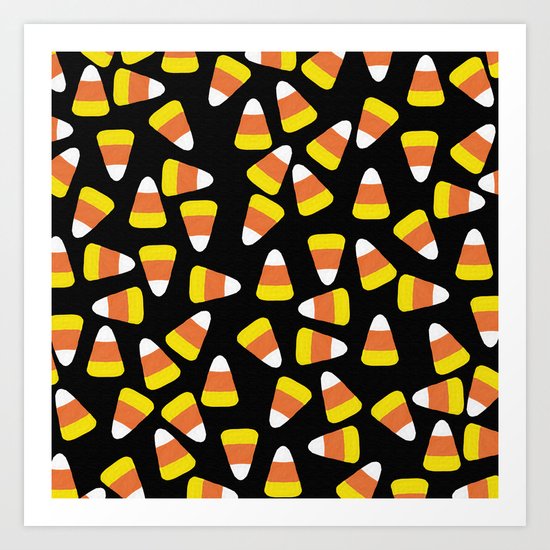This image showcases a graphic representation of numerous candy corn pieces, arranged haphazardly against a solid black background. Each piece, true to traditional candy corn, features a white tip, an orange midsection, and a yellow base, all with rounded edges. The candy corn is oriented in various directions—up, down, and diagonal—spread unevenly but plentifully, with around 50 pieces in total. Surrounding the image is a distinct white border roughly an inch thick, which is further framed by a gray border. The clean design accentuates the scattered, vibrant candy corn against the stark black backdrop, creating a visually striking and festive composition.